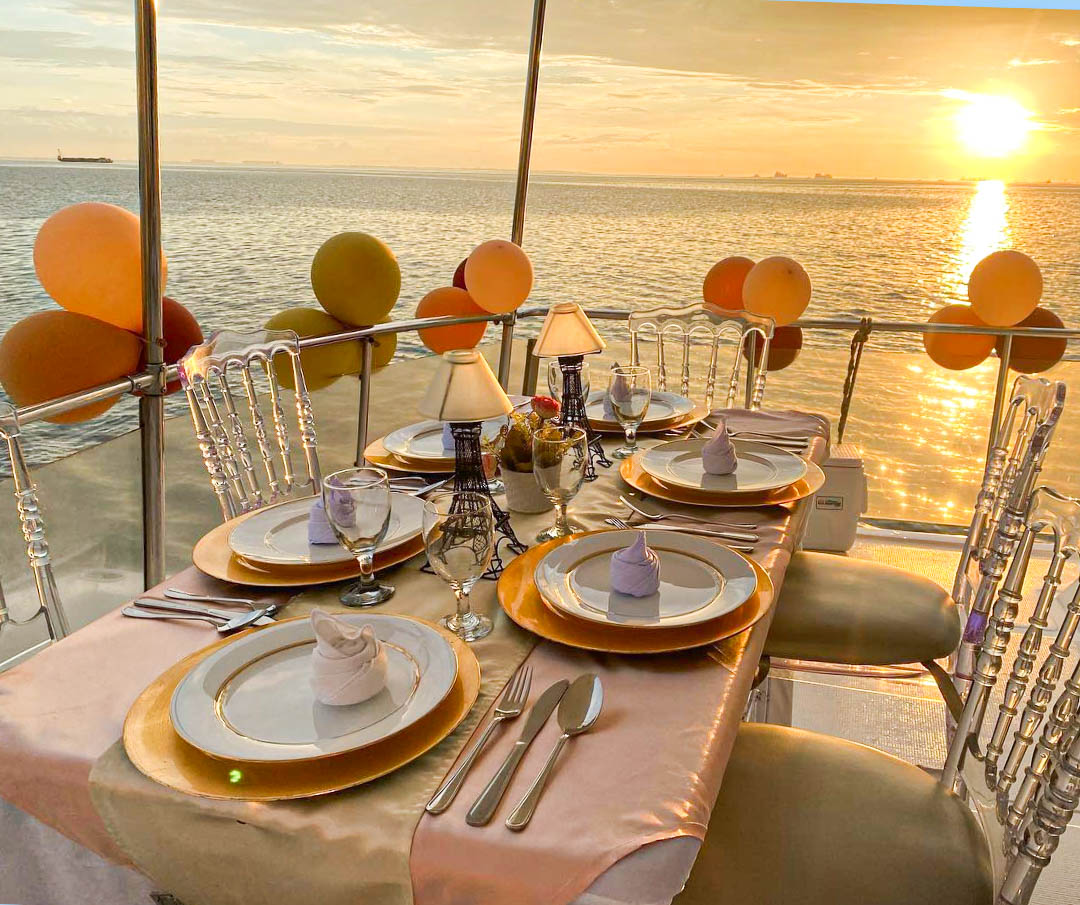The photograph showcases an elegant lakeside dining area at sunset, with a sophisticated table set for six but featuring only five visible chairs. The sky is a mesmerizing blend of orange and blue hues, with the golden sun casting a warm glow over the scene. The background reveals a vast body of water dotted with ships, a prominent freighter, and distant tall buildings. The dining setup includes a white tablecloth overlaid with a pink silky one, and a long beige runner at the center. Each place setting features a plate, a water glass, and elegantly arranged silverware, with napkins folded like roses. The table is adorned with two lamps with black bases, and the railing is decorated with bunches of orange and lavender balloons, enhancing the celebratory atmosphere.